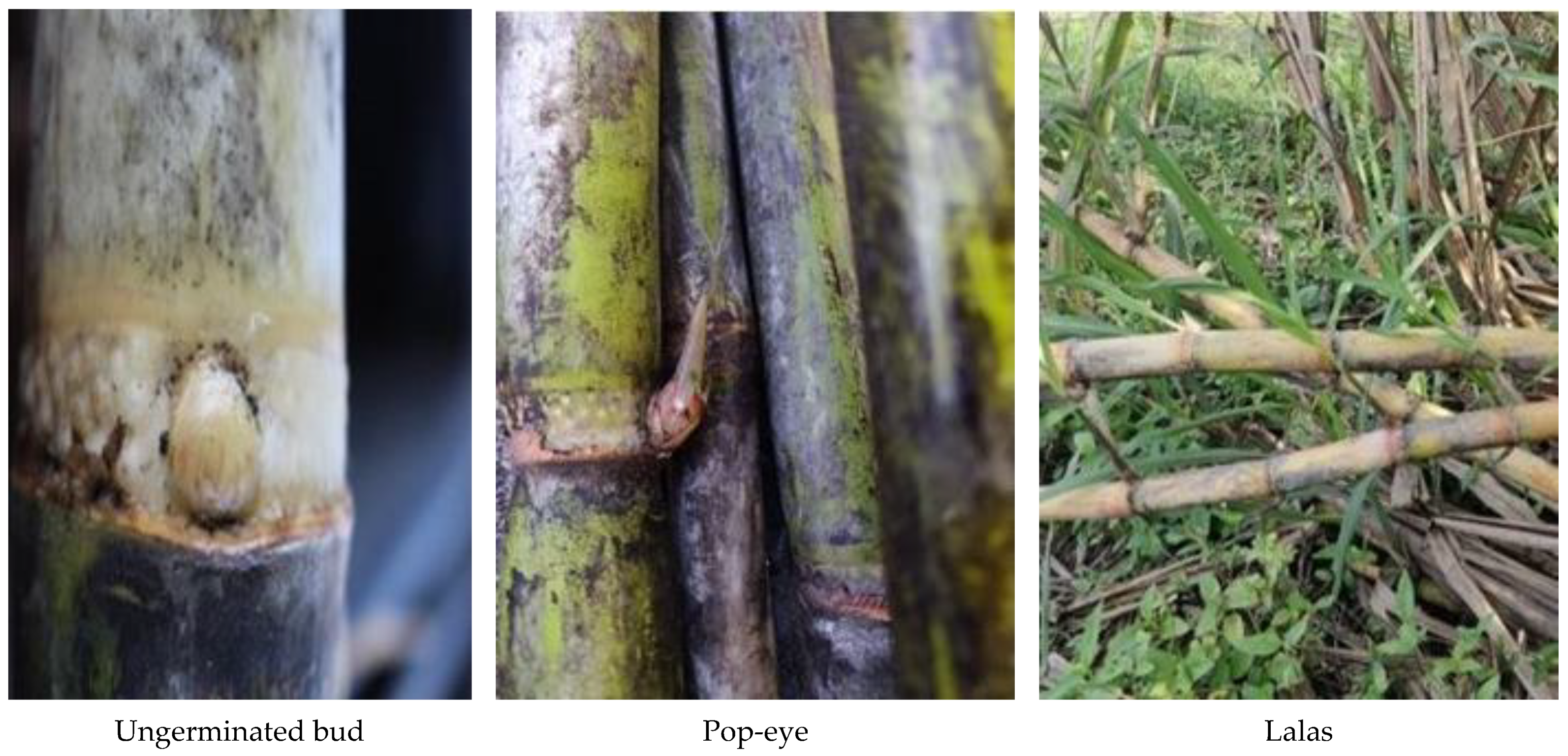The image comprises three side-by-side, low-quality photographs set against a white background. Each photograph features trees, likely bamboo, with accompanying text at the bottom. The first image, labeled "un-germinated bud," shows a close-up of a bud that appears in the center of a tree, resembling an egg in a tree, though details are difficult to discern. The second photograph, titled "Popeye," depicts an animal subtly peeking through the branches of a more deteriorated tree, blending seamlessly with the surroundings. The final image, labeled "lalas," presents a dense cluster of branches and leaves where an animal, even more camouflaged, can barely be detected. Collectively, these images highlight the theme of natural camouflage in wildlife.